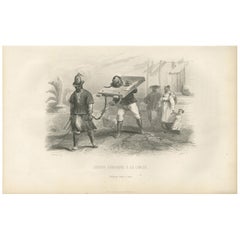The image is a vintage, sepia-toned illustration on weathered parchment-like paper, depicting a historical scene. At the center, a conquistador donning a smooth helm and robe-like armor is prominently displayed. He is pulling a chained native or slave, whose head and arms are confined within a rectangular wooden shackle, making escape impossible. This enslaved man, wearing white trousers, black boots, and a black shirt, appears to be struggling on a dirt path. In the background, an indifferent aristocratic couple observes the scene, while further back, a family with children and possibly some trees and houses are faintly visible. The edges of the paper are worn, and although there is a caption below the central illustration, it is blurred and unreadable.